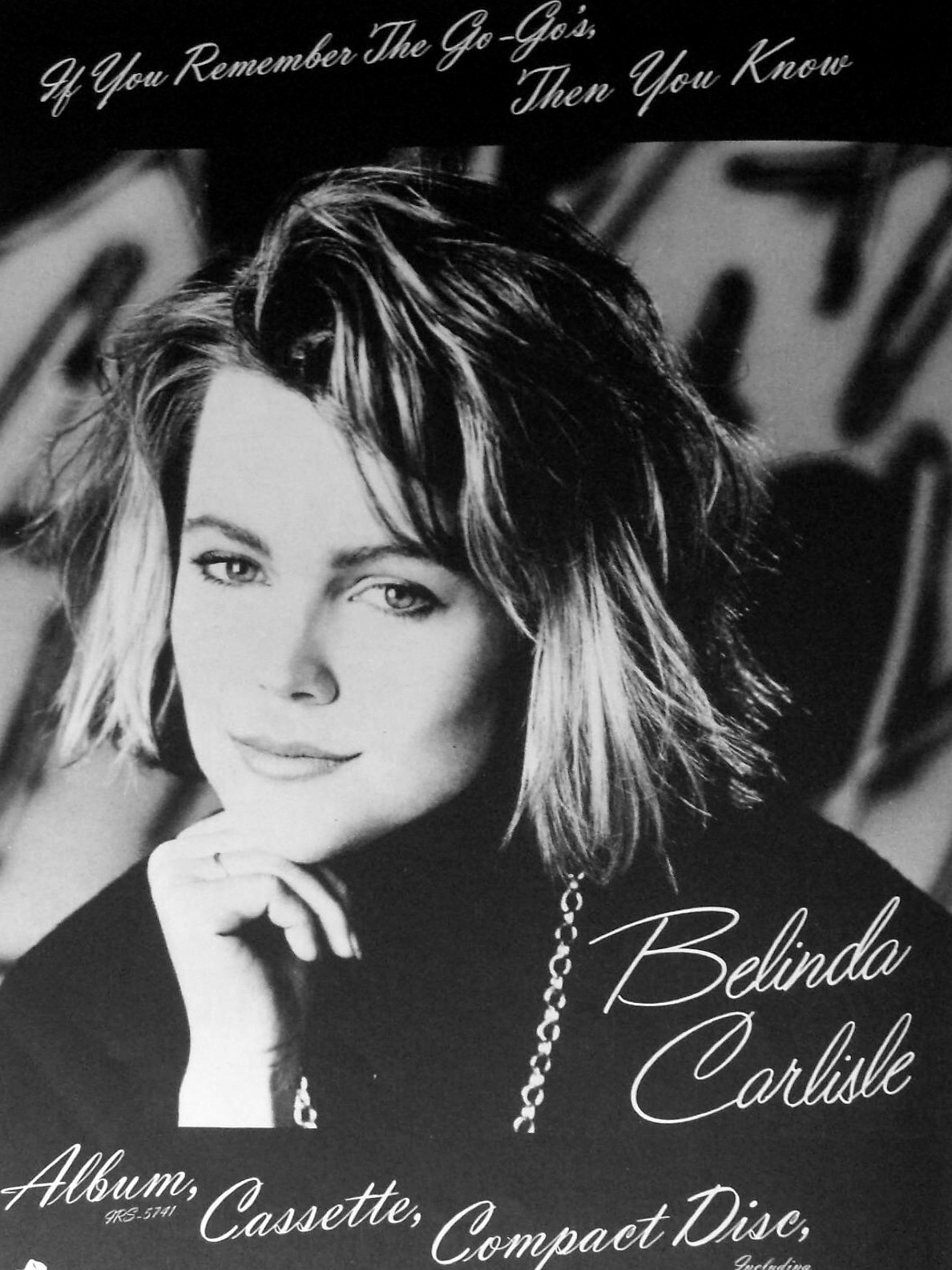In this black and white photograph, a youthful-looking Belinda Carlisle, likely in her mid to late 20s, is captured with her head tilted slightly clockwise, resting her chin on her fingers. She gazes thoughtfully towards the camera with a subtle, closed-mouth smile. Her shoulder-length hair is tousled and poofy, adding a touch of messiness to her look. She dons a dark black top accentuated by a bold, thick chain necklace. On her ring finger, a ring is visible. 

The background is a blend of indistinct black and white patterns, reminiscent of graffiti art, adding an edgy vibe to the image. Handwritten at the top in cursive is the phrase, "If you remember the Go-Go's then you know." At the bottom right, her name "Belinda Carlisle" is printed in italics. Further down at the bottom, it reads, "album SRS 5741 cassette compact disc," suggesting promotion for her music through various formats.